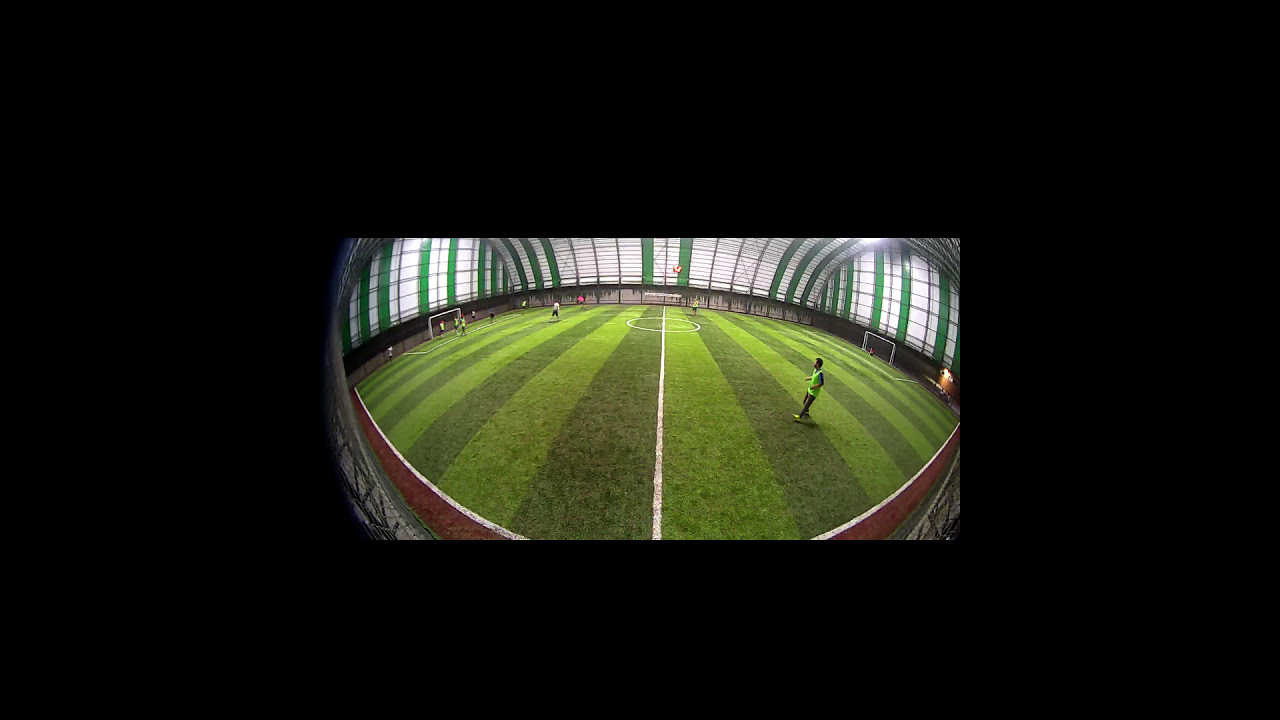This is a 360-degree panoramic image of an indoor soccer field, taken with a fisheye lens, giving it a distinctive curved appearance. The field features a striking checkered pattern of alternating dark green and light green grass. In the center, a white line bisects the field, leading to a central circle, characteristic of a soccer pitch. Dark brown dirt borders the field, curving up around the edges.

In the foreground, to the right, a person stands wearing a green tank top and long pants. This individual appears to be running. There are several other players scattered across the field but mostly clustered near the left goalpost, dressed randomly without uniforms.

The background reveals green and white striped walls, allowing some natural light to filter through, suggesting a partially transparent or glass structure. The roofing, also checkered with white and green glass, spans the entire stadium. Additionally, nets flank either side of the image, indicative of the goal areas. No crowd is visible, emphasizing the solitary feel of the scene.